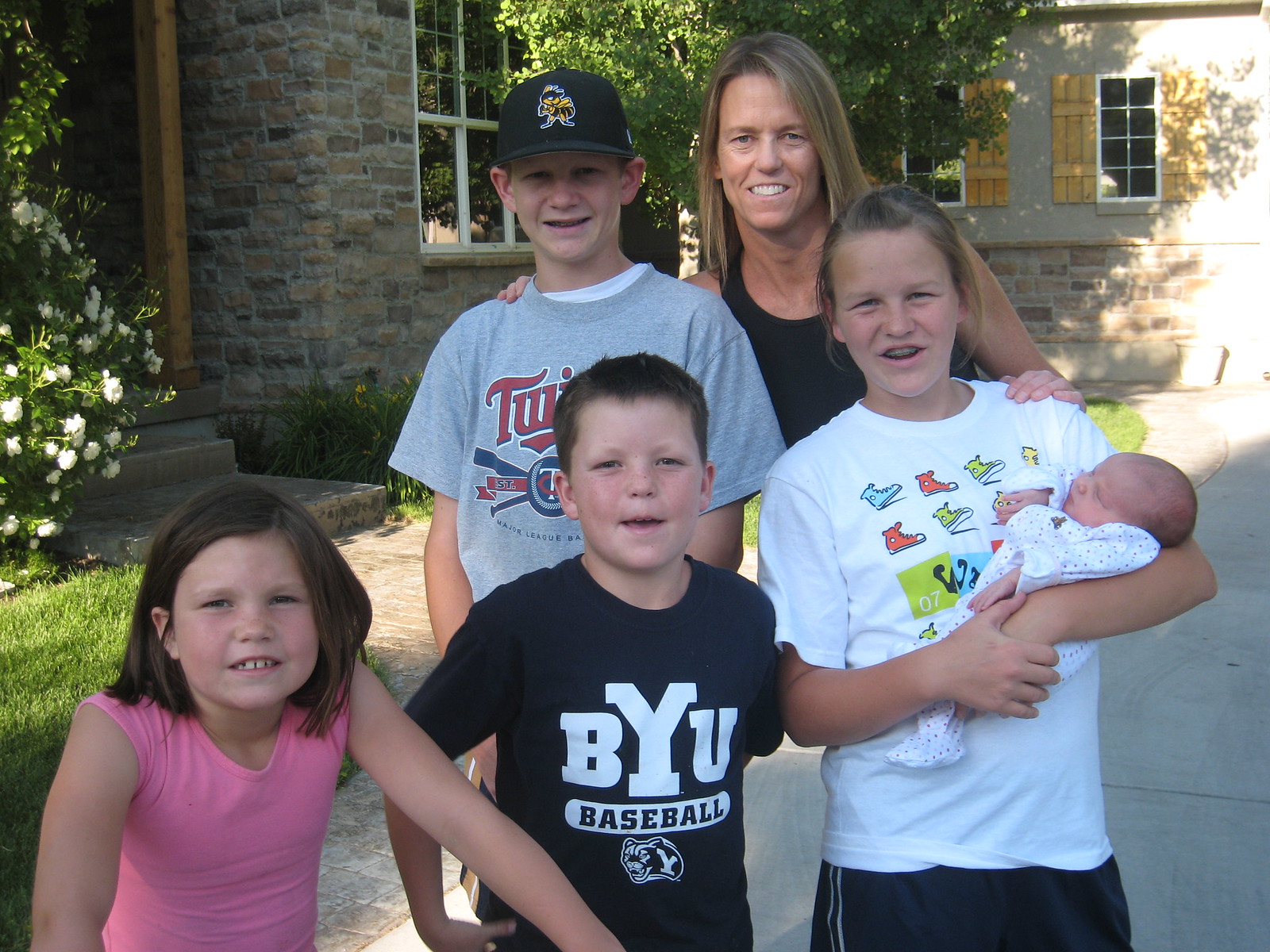This is a detailed family photo taken outdoors in what appears to be a driveway or walkway in front of a home, visible in the background with its windows and yellow shutters. Flower bushes and a small tree add a touch of greenery and vibrance in front of the house. 

The family consists of six people – a woman who appears to be in her 40s with light brunette hair standing towards the back, and four children along with a tiny newborn baby. The children are dressed in short sleeves, indicating it's a warm and sunny day. 

On the left, a smiling little girl is wearing a pink tank top. Next to her, a young boy at the front is dressed in a blue BYU baseball t-shirt. Behind him stands an older boy wearing a gray Twins t-shirt and a baseball cap. To the right, another girl, who has her hair pulled back and is wearing blue athletic shorts and a t-shirt, is tenderly holding the newborn baby, who is dressed in a white baby outfit and appears to be just a week or two old. 

The mom, standing with a sleeveless tank shirt, smiles warmly at the camera, capturing a joyful and loving family moment.